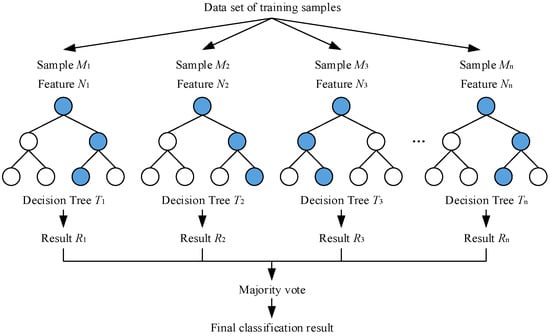The image depicts a detailed educational schematic in black, white, and blue colors, representing the flow of training samples through a classification process. At the top, the schematic is labeled "Data Set of Training Samples," with arrows pointing to four columns labeled Sample M1 (Feature N1), Sample M2 (Feature N2), Sample M3 (Feature N3), and Sample MN (Feature NN). 

Below these samples, there are interconnected circles illustrating combinations of blue and white dots, each corresponding to the respective samples. These combinations lead to the formation of decision trees for each column, labeled Decision Tree T1, Decision Tree T2, Decision Tree T3, and Decision Tree TN. 

Four downward-pointing arrows emanate from these decision trees, each resulting in outcomes labeled Result R1, Result R2, Result R3, and Result RN. These results are collectively fed into a majority vote mechanism, culminating in a final arrow that indicates the final classification result. 

This entire flowchart presents a structured representation of a data classification process, likely part of an academic or educational resource.